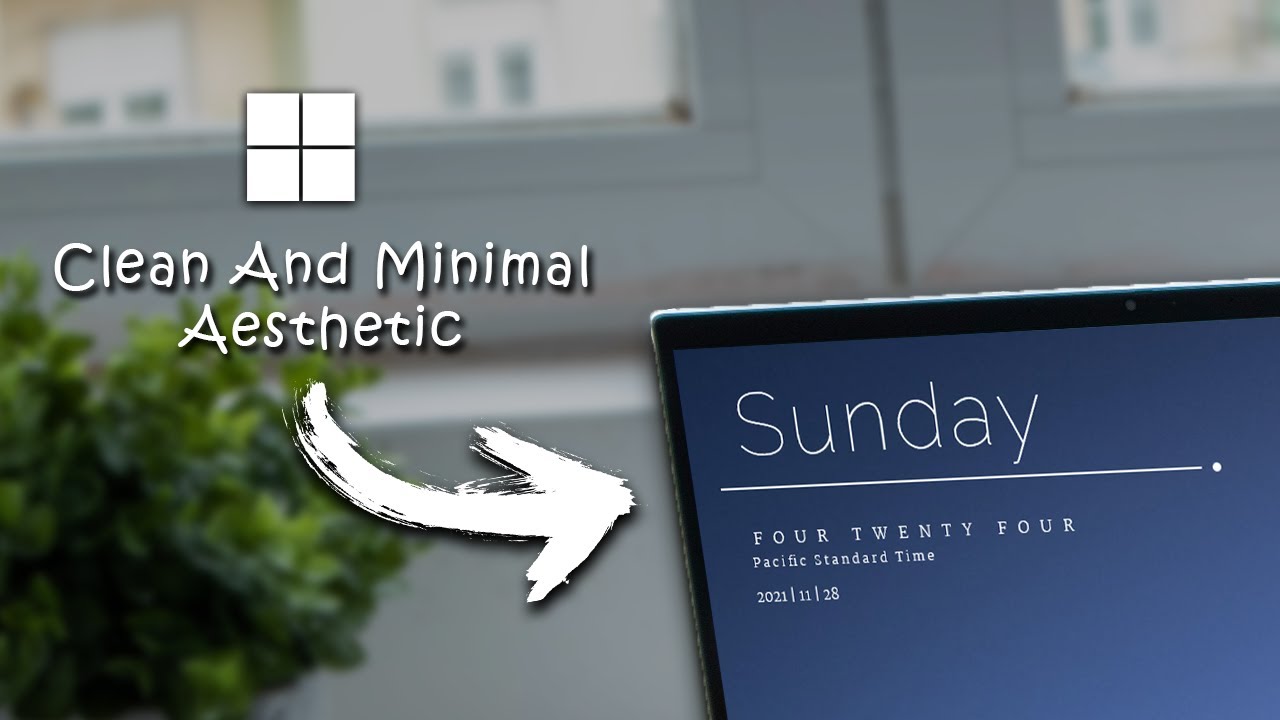The photograph features the top portion of an opened laptop screen in focus, set against a slightly blurred background that includes white windows and a green potted plant on the bottom left. On the laptop screen, "Sunday" stands out in large, underlined white letters against a blue background. Below it, written in smaller white text, it says "4-24 Pacific Standard Time, 2021/11/28," all spelled out in letters. To the left of the screen, there is a white square with a cross-like symbol inside it. Below this icon, the phrase "Clean and Minimal Aesthetic" is written in white against a gray background, accompanied by a rough, brushstroke-style arrow pointing towards the laptop screen from the upper left to the bottom right, emphasizing the screen’s content. The overall composition suggests a modern and uncluttered aesthetic.